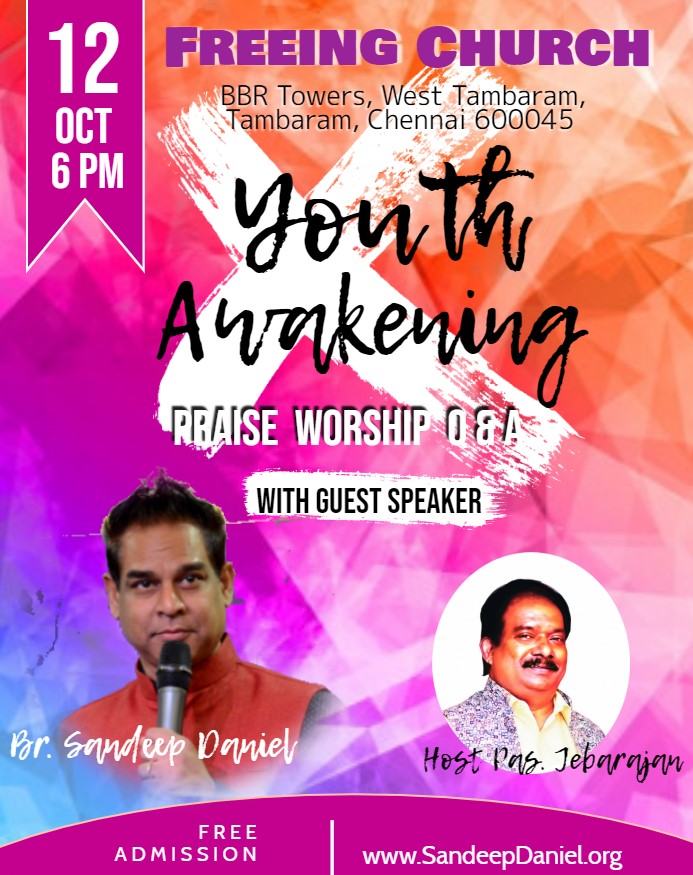The advertisement is a vibrant flyer for a church gathering hosted by Freeing Church at BBR Towers, West Tambaram, Chennai, 60045. The event, titled "Youth Awakening," is scheduled for 12th October at 6 PM and features a lineup of Praise, Worship, and Q&A sessions. The colorful background blends hues of blue, magenta, purple, pink, and orange, with geometrical patterns enhancing the visual appeal. A prominent white cross is centered on the flyer, symbolizing the religious nature of the event. Just below the church's name at the top, the venue details follow in black font. The event title, "Youth Awakening," is artistically written in cursive, overlaid on the cross. Below this, in white font, the activities "Praise, Worship, Q&A" are listed. The flyer features photos of two men at the bottom: on the left is Sandeep Daniel, identified as the host, and another guest speaker on the right, though his name is less legible. The bottom of the flyer states "Free Admission" and provides a website, www.sandeepdaniel.org, offering additional details. A ribbon graphic on the left side marks the date and time of the event.